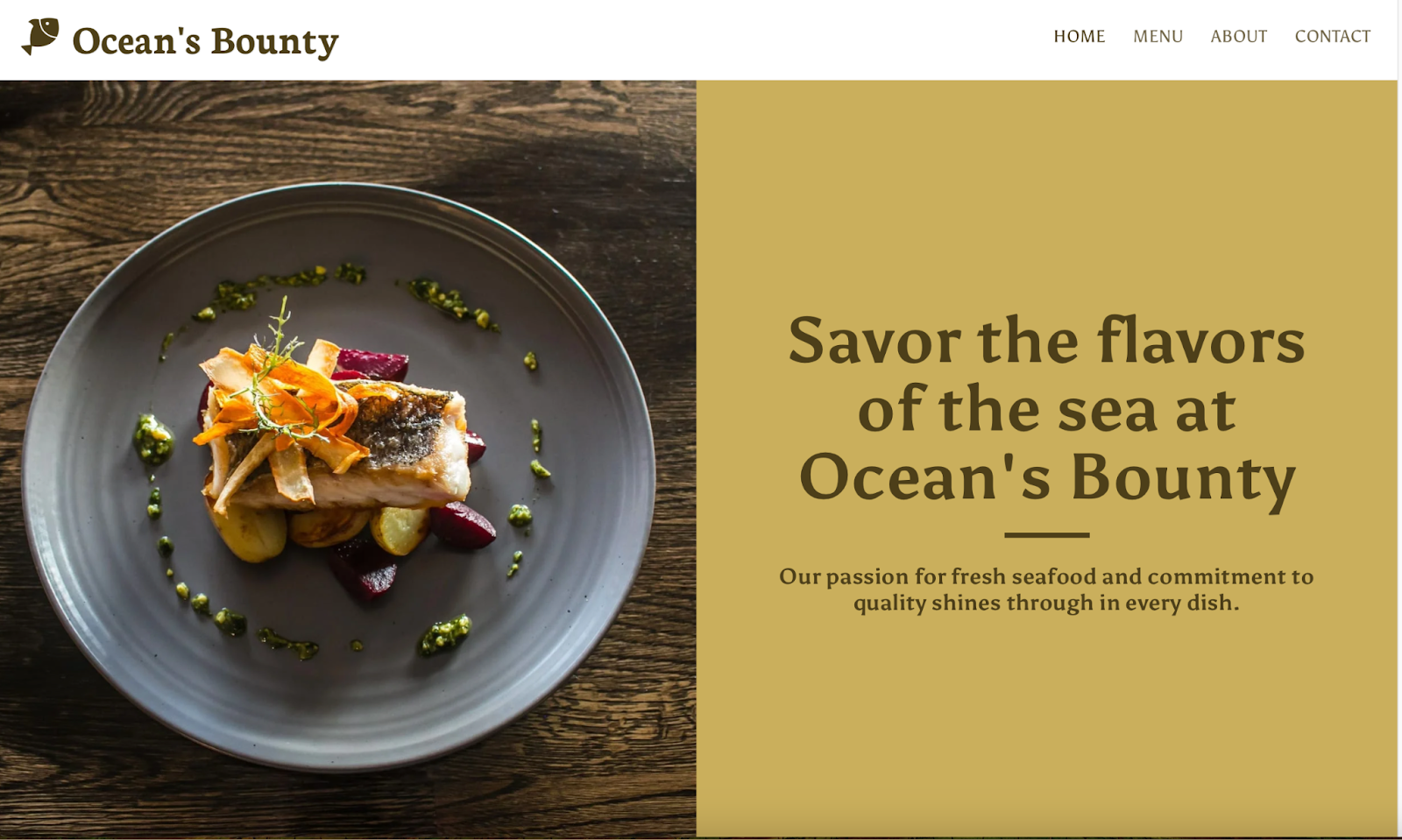In the upper left corner of the image, "Ocean's Bounty" is prominently displayed in brown text, accompanied by an icon of a fish. The background of this upper section is white. To the top right, four navigation tabs—Home, Menu, About, and Contact—are also written in brown.
The right half of the image features a light brown background with a darker brown inscription that reads: "Savor the flavors of the sea at Ocean's Bounty. Our passion for fresh seafood and commitment to quality shine through in every dish."

Centrally positioned on the right side and spanning the left half of the image is a round, slightly gray plate set on a wooden table. The table’s brown surface showcases darker wood grain textures. The plate's presentation is eye-catching: a green sauce mixture is artfully drizzled in a circle around its perimeter. Within this circle, various elements of a seafood dish are arranged. The seafood itself boasts brown, white, and dark hues, accented with red elements and topped with a sprig of green plant. To finish, there are yellow peels delicately placed atop the dish, offering a vibrant contrast.